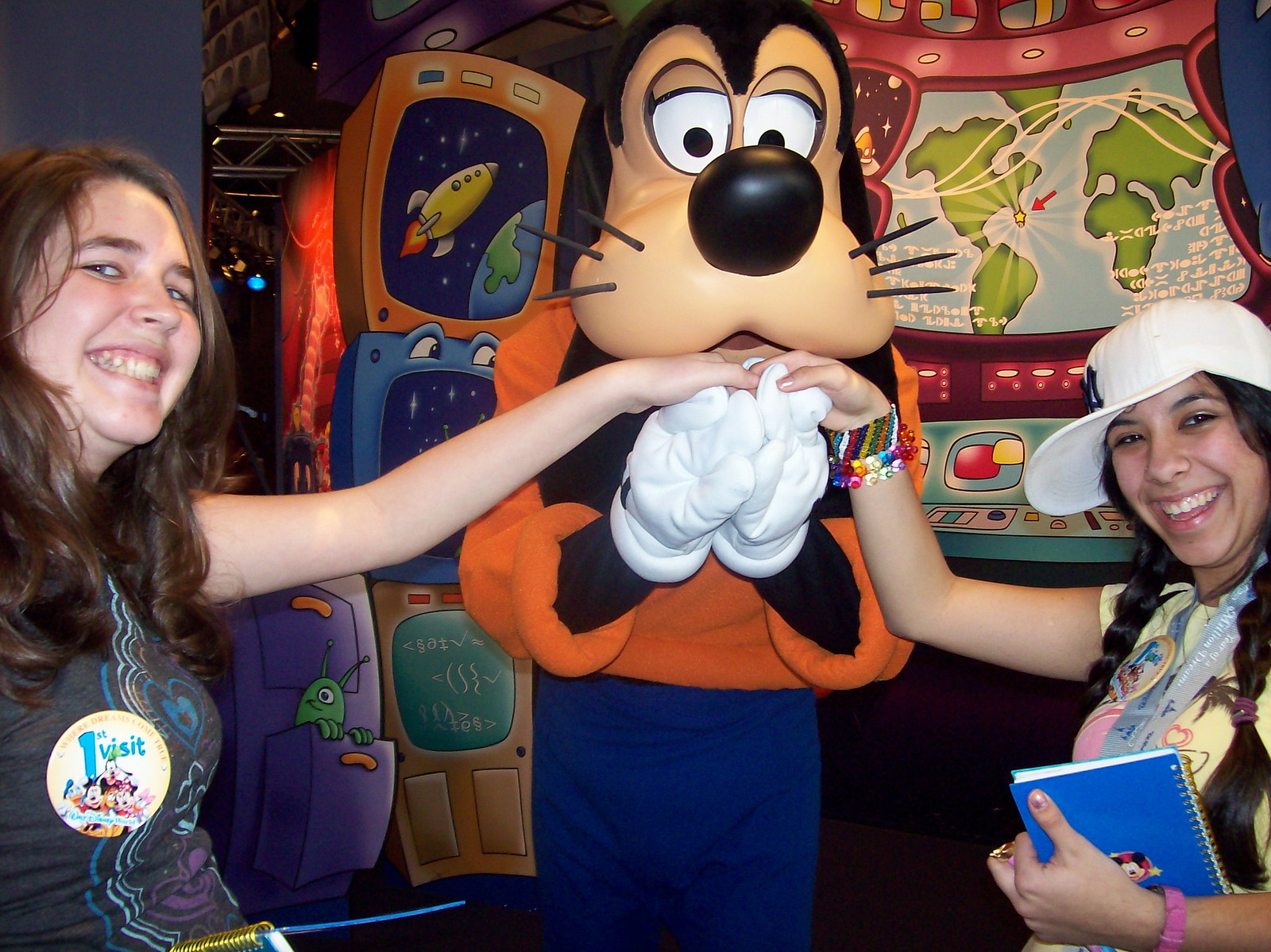The image depicts a lively indoor scene, presumably at Disney World, centered around a person dressed as the Disney character Goofy, who is wearing blue pants and an orange and black top. Surrounding him are two smiling women, both Caucasian and holding Goofy's hands—one on either side. The woman on the right is adorned with a white baseball cap and long braids, wearing a yellow graphic t-shirt, and is holding a blue spiral notebook with a brown cover in her left hand. She also sports numerous bracelets, including a pink one on her left arm. The woman on the left, with long dark hair, is dressed in a gray t-shirt and is wearing a button that reads "First Visit" featuring images of Mickey Mouse and Minnie Mouse. The backdrop includes a vibrant cartoon-like display reminiscent of a spaceship, filled with colorful lights and intricate designs, adding a whimsical touch to the joyful atmosphere of the arcade-like setting.